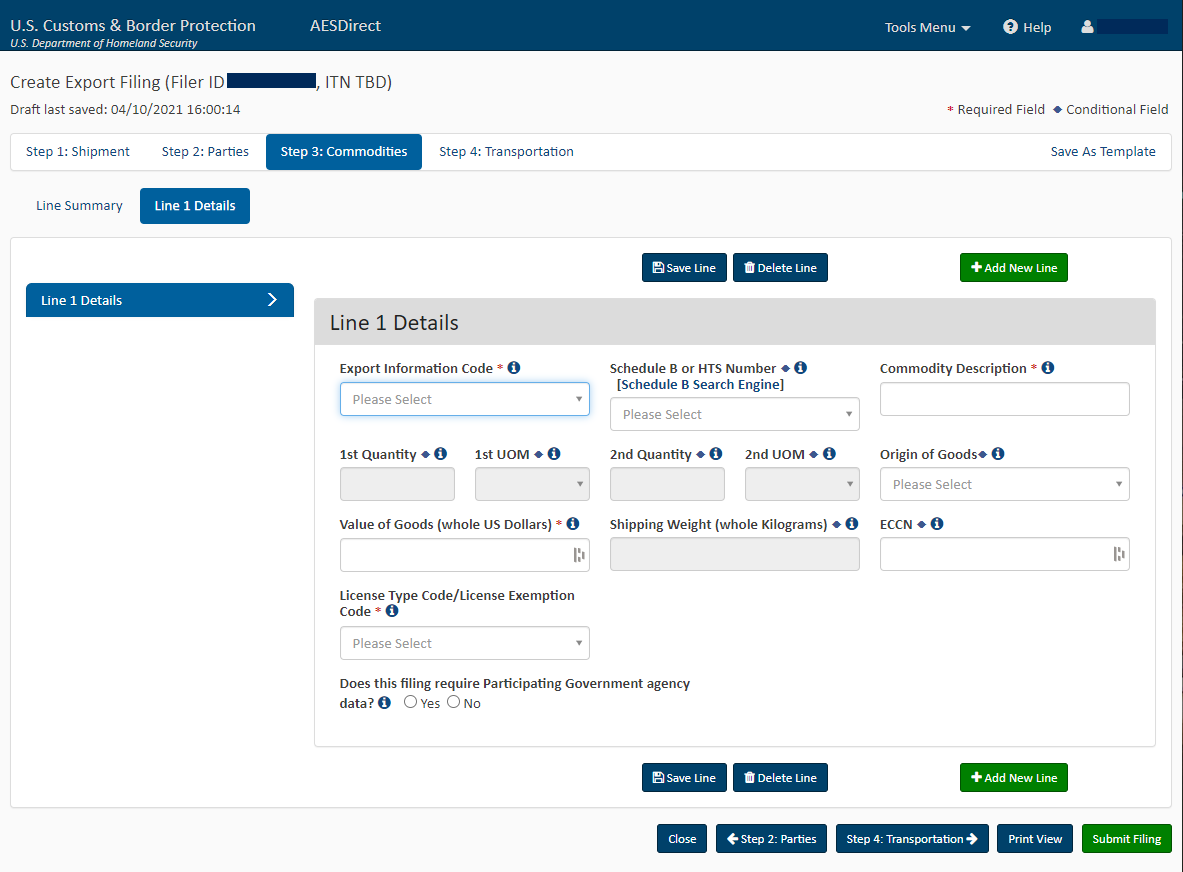This screenshot displays the user interface of the U.S. Customs and Border Protection's AES Direct portal, managed by the U.S. Department of Homeland Security. The top-left corner features the official logos of these agencies. Adjacent to this, the interface includes a navigation bar with a "Tools" dropdown menu, a help shortcut indicated by a question mark, and a sign-in button represented by a profile icon.

Prominently positioned below the navigation bar is the main action button labeled "Create Export Filing," alongside a masked Filer ID and an ITN status listed as "TBD" (to be determined). Further below, the screen notes the draft's last save date as April 10, 2021, precisely at 16:00:14 hours.

The interface is divided into a series of steps, visible as tab labels: Step 1 - Shipment, Step 2 - Parties, Step 3 - Commodities, Step 4 - Transportation, and a "Save As Template" option. The highlighted tab indicates the user is currently in Step 3 - Commodities, which is shaded in blue.

The section beneath the highlighted tab reads "Line Summary" with a focus on "Line 1 Details." This area contains numerous input fields essential for export documentation: Export Information Code, Schedule B or HTS Number, Commodity Description, Origin of Goods, and Value of Goods (in US dollars). There is also an ECCN field (Export Control Classification Number) and a section for License Type Code or License Exemption Code.

Towards the bottom of the form, a question asks whether the filing requires data from a participating government agency, with corresponding 'Yes' and 'No' radio button options available for selection.